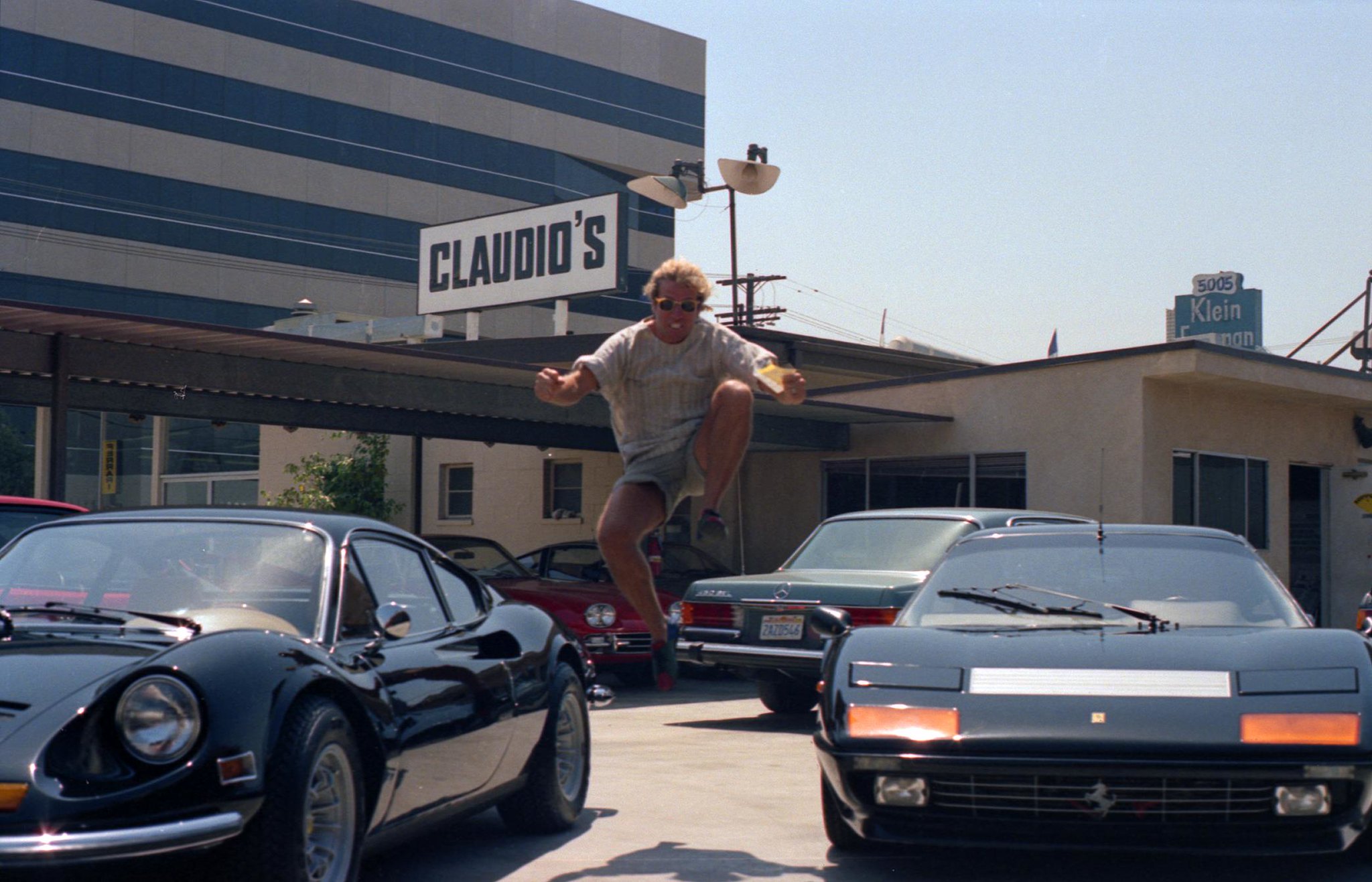In this color landscape photograph, a man is captured mid-leap between two parked sports cars in a parking lot under a clear, light blue sky. The central figure is a smiling man with blonde curly hair, wearing sunglasses, a light gray t-shirt, and cutoff blue jean shorts. He is suspended about three feet in the air, facing the viewer with his left knee bent towards his chest and arms spread wide. On his left is a rounded sport car with dark blue or black paint, resembling a Porsche, and on his right is another dark sports car featuring distinctive orange running lights and a central white light strip. Behind this setup, a small single-story beige building with a prominent black and white billboard that reads "Claudio's" is visible. Further in the background, a partially obscured sign on a taller building reads "Saad's Klein." The scene blends photographic realism with a sense of dynamic movement.